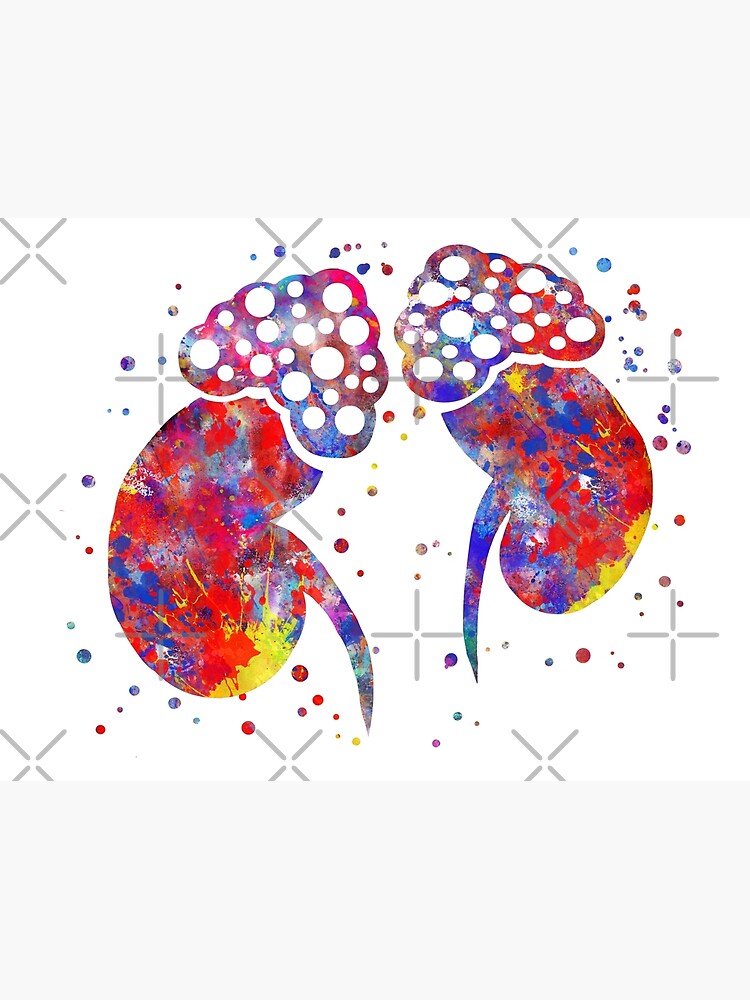The image depicts a pair of kidneys with a background featuring gray cross patterns and multicolored dots in shades of purple, red, blue, and yellow. Each kidney is adorned with a cloud-shaped section at the top, containing large and small white circles against a vibrant background of red, blue, and green. The lower sections are distinctly kidney-shaped, and within each kidney, there is a tail-like structure emerging. The entire composition is accentuated with splashes of blue, red, and yellow, giving it a dynamic and artistic appearance suggestive of a splatter paint effect.